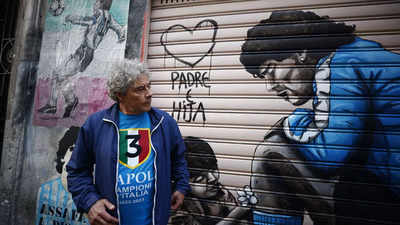In this image, the side of a street building is adorned with vibrant mural art. At the center, the mural features a black man with curly hair and earrings in his left earlobe, dressed in a blue jersey with white stripes on the sleeves. He is hunched over on his knees with his eyes closed, facing a child who is offering him a flower. To the left of this heartfelt scene, written in black spray paint, is the phrase "Padre Ahija" along with a heart symbol. 

In front of the mural stands an older gentleman with silver curly hair. He wears a bright blue sporting jersey that bears the emblem of a flag in green, white, and red, alongside the text "Apole Champion Italia." Over his jersey, he has on a darker blue windbreaker. Further to the left of the man and the central mural, more artwork is visible on the building’s wall, including the depiction of a soccer player in action.